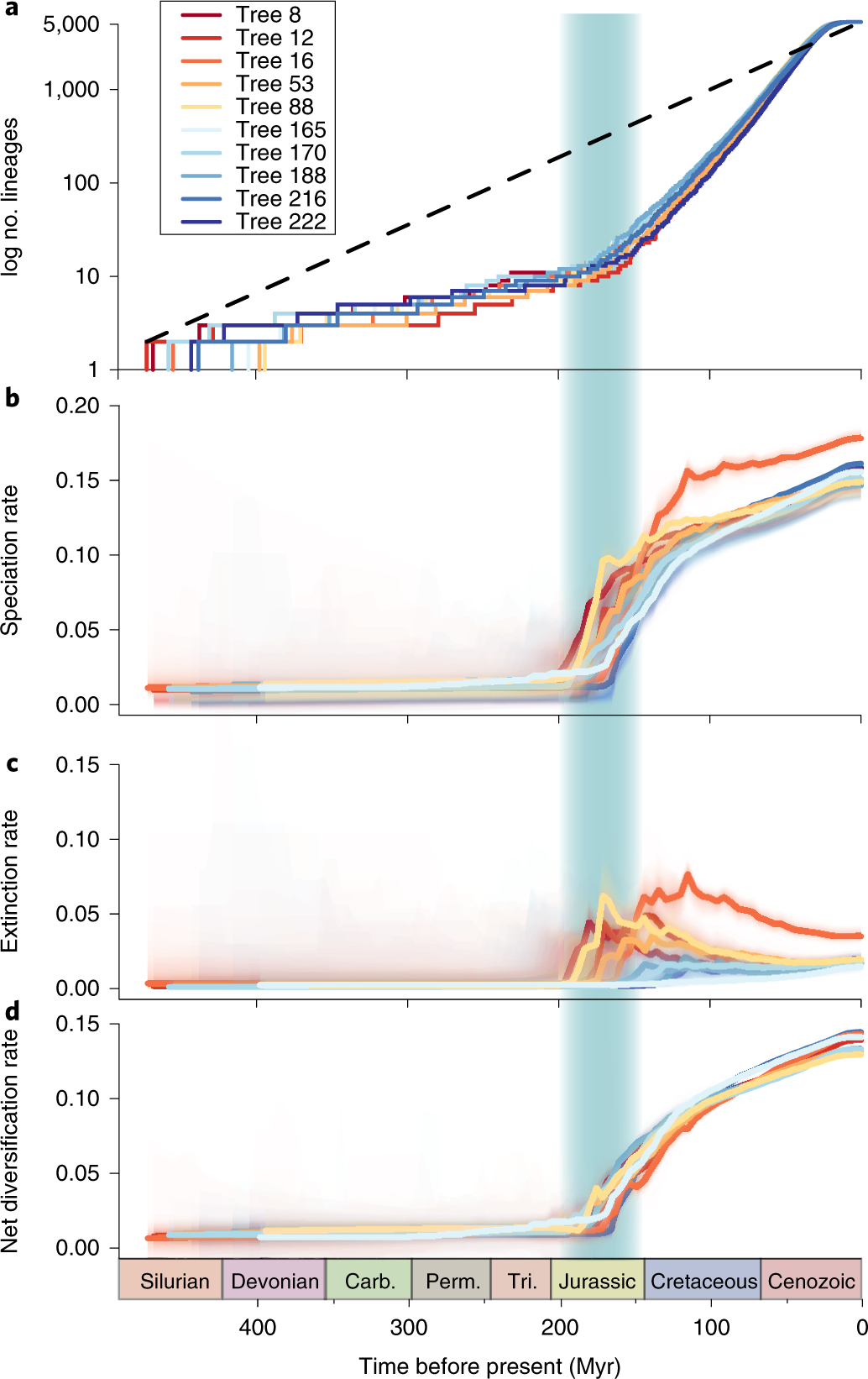The image features a vertical rectangular informational chart with a white background, comprising four horizontal sections stacked one on top of the other, each wider than it is tall. Each section represents a different metric over time: 

1. Section A at the top shows the "Log Number of Lineages."
2. Section B shows the "Speciation Rate."
3. Section C presents the "Extinction Rate."
4. Section D at the bottom indicates the "Net Diversification Rate."

The y-axis on the left side of each section is marked with these respective labels, and they all share a common x-axis at the bottom representing geological time periods, labeled from left to right: "Silurian," "Devonian," "Carboniferous (Carb)," "Permian (Perm)," "Triassic (Tri)," "Jurassic," "Cretaceous (Cretaceous)," and "Cenozoic." The x-axis also includes a timeline indicating "Time Before Present" with markers at 400 MYR (Million Years Ago) through to 100 MYR.

Each section features multiple colored lines, each representing different trees, denoted by "Tree" followed by numbers such as Tree 8, Tree 12, Tree 16, and so on up to Tree 222. The lines generally start from the bottom left corner, gradually rising and then sharply increasing halfway through the chart, moving up and to the right.

Additionally, there is a smaller inset chart located in the upper left quadrant of the image, showcasing various colors correlated with specific tree numbers. The entire chart is well-labeled to convey how these different metrics have evolved over significant prehistoric time periods.